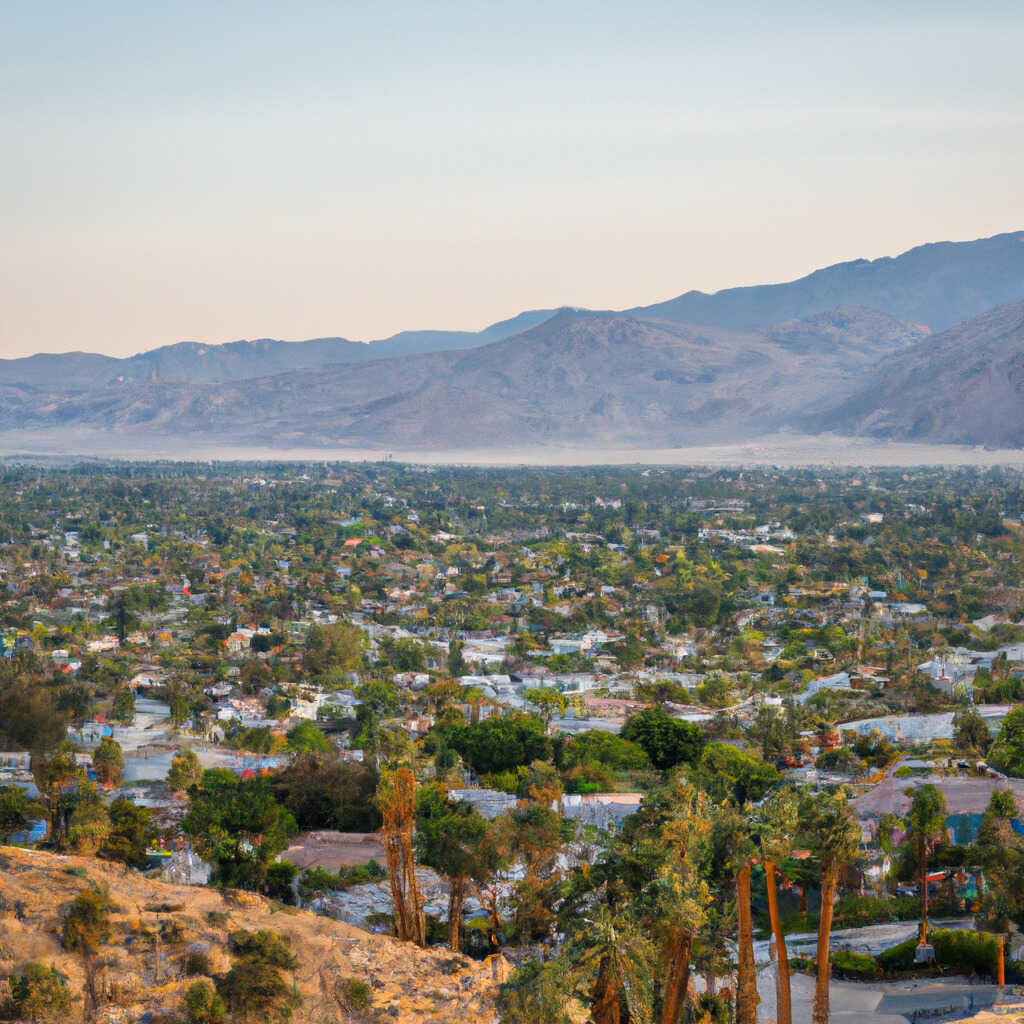This color photograph captures a serene, suburban community nestled in a desert-like valley. The foreground features a rocky outcropping with scattered bushes, leading to single-dwelling homes with possible Spanish-tiled roofs. These homes, intermixed with lush palm trees and varying foliage, paint a peaceful scene. The suburban landscape is dotted with backyard pools and intertwined by roads, though the exact details are indistinct due to the image's resolution. Looming in the background are impressive mountains, sparsely vegetated and forming a gradual ascent from left to right. The sky, transitioning from a soft pink near the horizon to a light blue at the top, suggests it's early morning, infusing the scene with a tranquil, waking-up ambiance. The entire setting evokes a feeling reminiscent of places like Palm Springs.